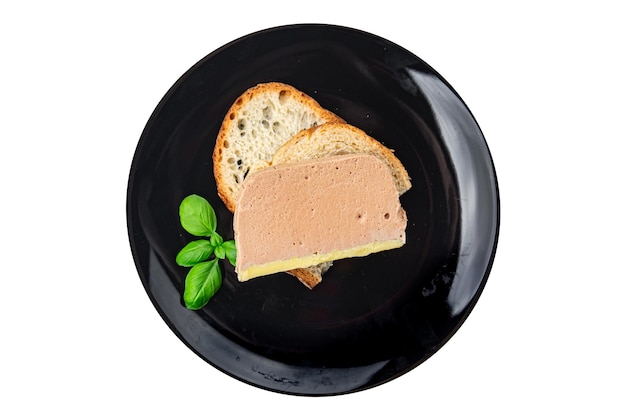The image displays a top-down view of a shiny, round black plate on a white background. On the plate are two flaky, airy slices of crusty French bread with a brown crust and white, hole-speckled interior. Partially covering the bottom slice is a pink piece of processed meat, possibly liverwurst, with a flat bottom, rounded sides, and a noticeable yellow strip along the bottom edge which may be seasoning, fat, or butter. The meat also has a few speckles and a porous texture. To the left of this arrangement is a light green sprig of basil, bearing six leaves, adding a fresh touch to the presentation. The plate itself has areas of shine on the right side and bottom left, enhancing its sleek appearance.